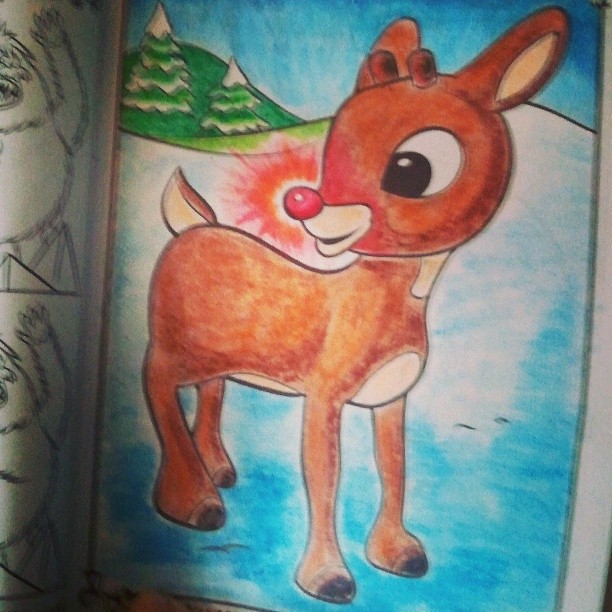This image showcases an open coloring book featuring a detailed rendition of Rudolph the Red-Nosed Reindeer inspired by the classic 1950s Christmas movie. The artist has skillfully colored the scene, with meticulous attention to detail. The snow is depicted in white and blue, adding a frosty, wintery touch. In the background, two decorated Christmas trees contribute to the festive atmosphere. Dominating the center of the page is a large, youthful Rudolph with his iconic glowing red nose, which the artist has enhanced with radiant sparks to emphasize its glow. Rudolph is depicted smiling, his expressive black eyes and warm brown fur capturing a joyful demeanor. His hooves are colored black, and he has budding antlers that hint at future growth. Additionally, his ears are decorated with darker brown on the outside and tan in the middle, contributing to the overall vibrancy and charm of this well-crafted holiday scene.